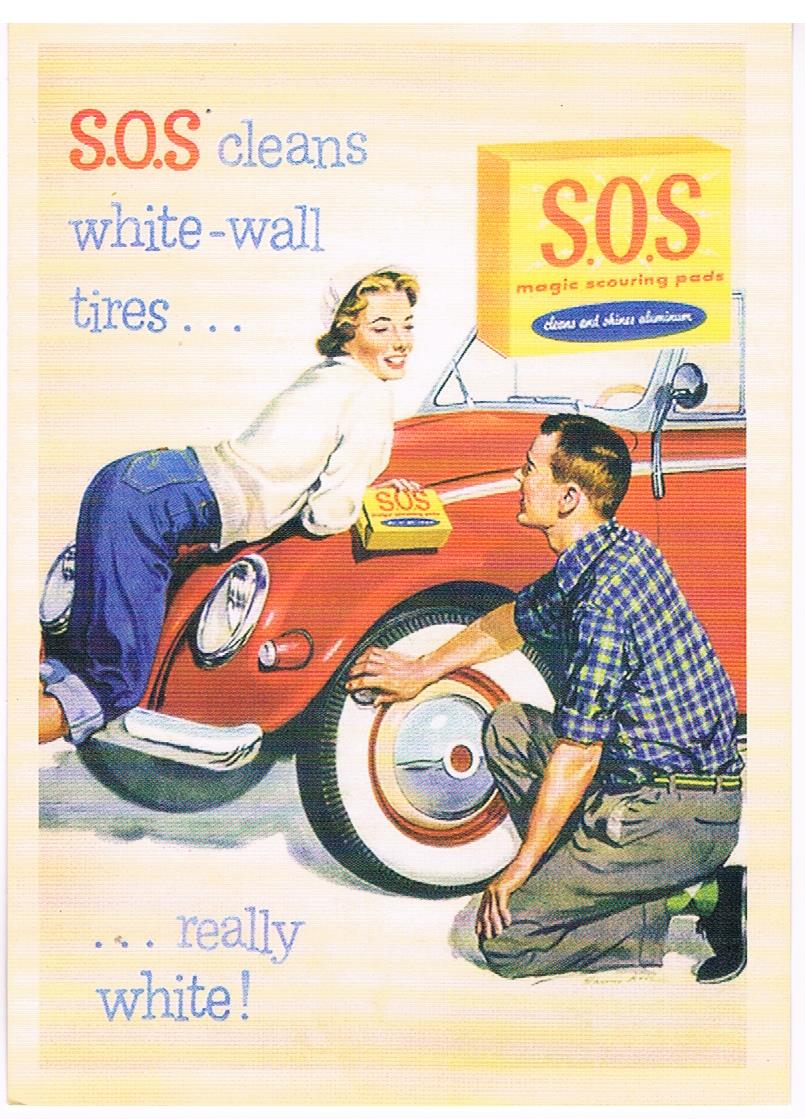The image appears to be a vintage advertisement, possibly from the 1950s, promoting SOS Magic Scouring Pads. The background is a soft pink hue, setting a nostalgic tone. Central to the image is a red Volkswagen Beetle, around which the scene unfolds. A blonde woman, dressed in a white long-sleeved top and rolled-up blue jeans, is leaning over the car's front hood, with her knees touching the chrome bumper. She holds a yellow box labeled SOS Scouring Pads in her right hand. Her white hat and smiling expression add to her vibrant appearance.

Beneath her, a young man with yellowish-reddish hair is kneeling at the lower right corner, intently scrubbing the car’s whitewall tire with a sponge. He is attired in a blue plaid shirt and gray pants, emphasizing the casual dynamic of the scene. The tire he’s working on is notably white, underscoring the effectiveness of the advertised product.

Across the top of the image, bold red and blue lettering reads, "SOS Cleans White Wall Tires," with "Really White" featured in the bottom left corner. Additionally, a large depiction of the SOS product box is prominently displayed in the upper right corner, further emphasizing the brand. The overall aesthetic and detailed drawings highlight the product's promise of cleanliness and efficiency.